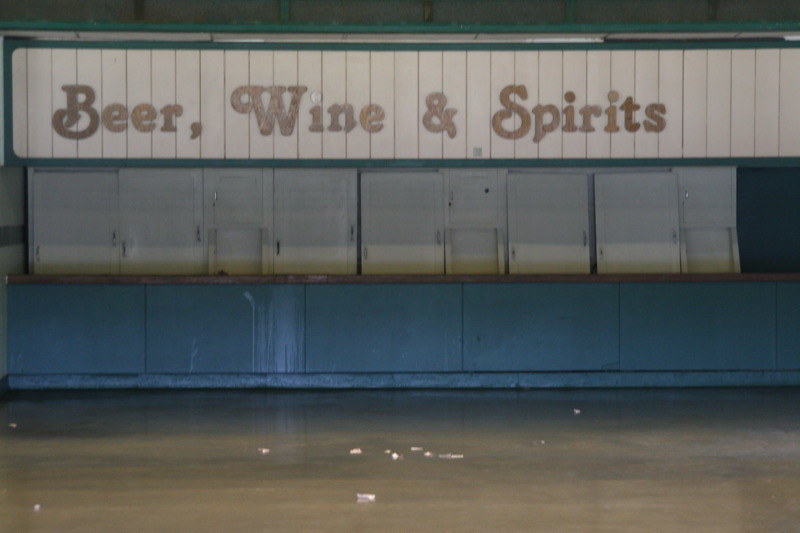The image depicts a seemingly abandoned concession stand situated along a road. The foreground features a road bordered by a blue-paneled barrier. Above the barrier, there's a horizontal array of approximately ten white doors or cabinets, suggesting storage or vending units. Above these doors, a large wooden paneled sign stretches horizontally, displaying "Beer, Wine, and Spirits" in old-style, gold lettering. The blue barrier below and white cabinets above it, combined with spilled liquids and scattered debris, give the impression that the area has not been in use for some time. The overall dilapidated appearance reinforces the notion that this concession stand is no longer operational.